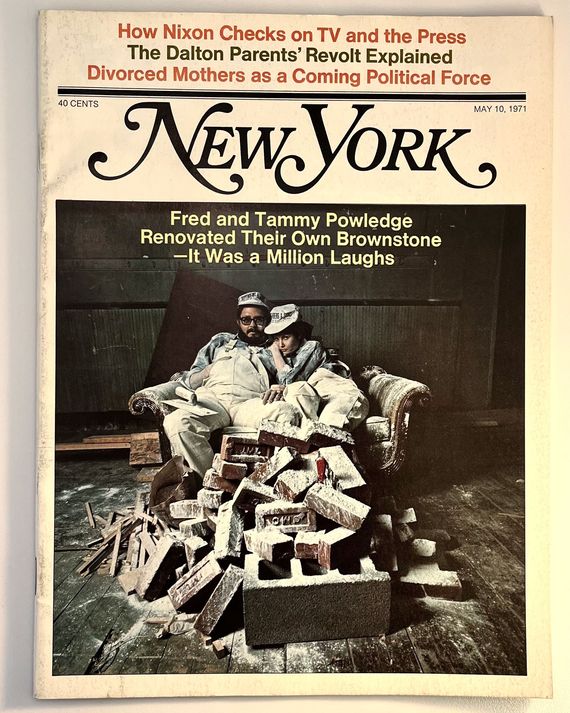This image showcases the cover of a vintage "New York" magazine dated May 10, 1971, and priced at 40 cents. Set against a gradient background that transitions from gray to yellow, the cover features prominent headlines in varying colors. At the top, red text reads "How Nixon Checks on TV and the Press," followed by "The Dalton Parents' Revolt Explained" in black, and "Divorce Mothers as a Coming Political Force" in red below that. 

The magazine title "New York" is displayed in large, stylized letters with curling embellishments. Below the title is an engaging photograph of a man and a woman. Both individuals are dressed in white painter's overalls and blue shirts, seated on a Victorian-style loveseat. The woman is leaning her body toward the man, who leans back comfortably. Surrounding the couple are dusty bricks and concrete cylinders, adding to the scene's rustic ambiance. The wooden floor beneath them is also covered in white dust, contributing to the overall sense of renovation and hands-on labor. Above the photograph, the caption in white text reads, "Fred and Tommy Powledge renovated their own brownstone. It was a million laughs."